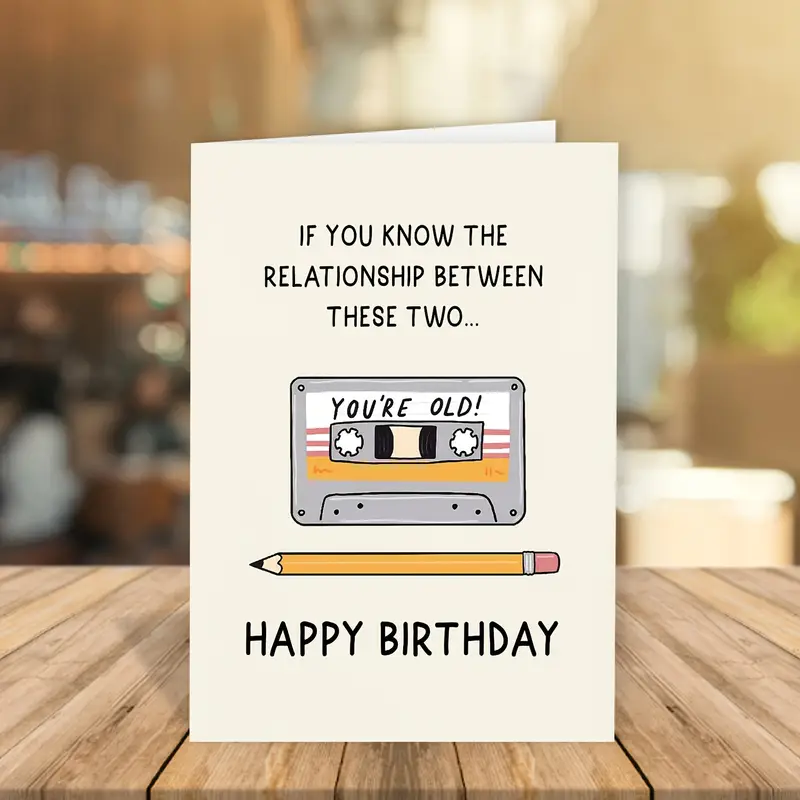The image depicts a birthday card standing upright on a brown wooden table. The card, which is a cream or off-white color, is slightly taller than it is wide and is partially open to the right, though its interior isn't visible. The front of the card features several elements: at the top, centered in black text, it reads, "If you know the relationship between these two..." Below this is a drawing of a gray cassette tape, which has the words "you're old" written on it in black. Underneath the cassette, there's a yellow pencil with a pink eraser, and just below the pencil, the card says "happy birthday" in black text.

The table on which the card stands has vertical light wood boards, and the background is out of focus, making details hard to discern. The background appears to be lit by natural sunlight from the upper right, possibly showing a lampshade and a variety of earth tones, including browns and blues, blending together. This nostalgic and humorous card can be appreciated by those who remember using a pencil to rewind cassette tapes, an activity hinted at by the design and text.